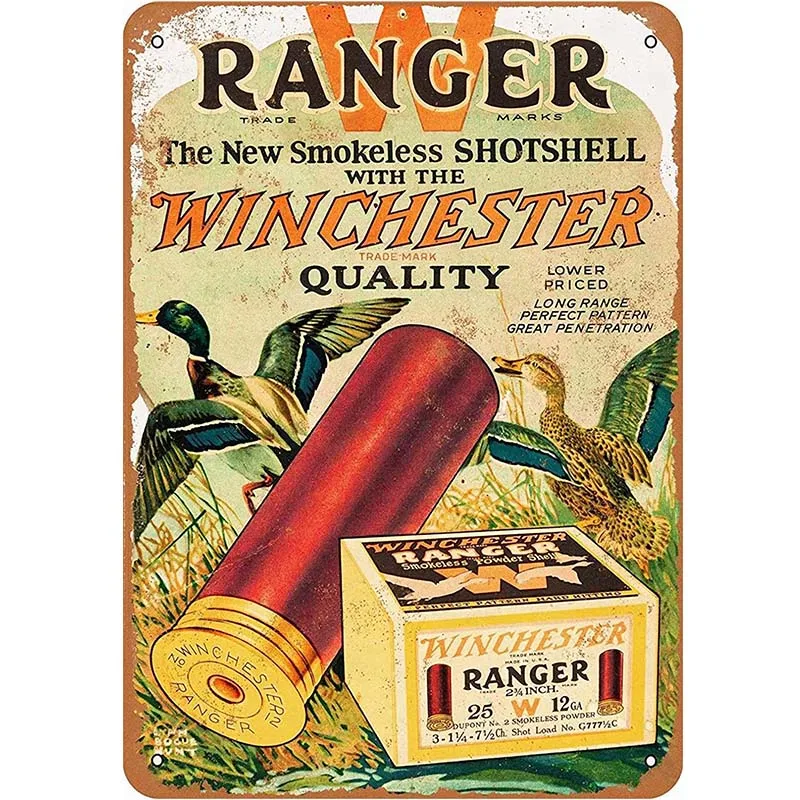This vintage advertisement for Winchester Ranger showcases the new smokeless shotgun shells with a nostalgic, worn graphic style typical of old Siamese advertising. At the top, the word "Ranger" is prominently displayed in curved black capital letters with an orange "W" behind it, signifying Winchester's trademark quality. The central image features ducks in the early stages of flight, emerging from a wet meadow with reeds, perfect for duck hunting. Dominating the lower section is a large red shotgun shell with a gold cap, labeled "Winchester Ranger." Beside this, a yellow box of the shotgun shells reveals packaging details. The entire sign, mounted with four drilled holes at the corners, displays notable wear around the edges, hinting at its age and authenticity. The advertisement emphasizes the shell's affordability, long range, perfect pattern, and great penetration, appealing to hunting enthusiasts seeking reliable ammunition.